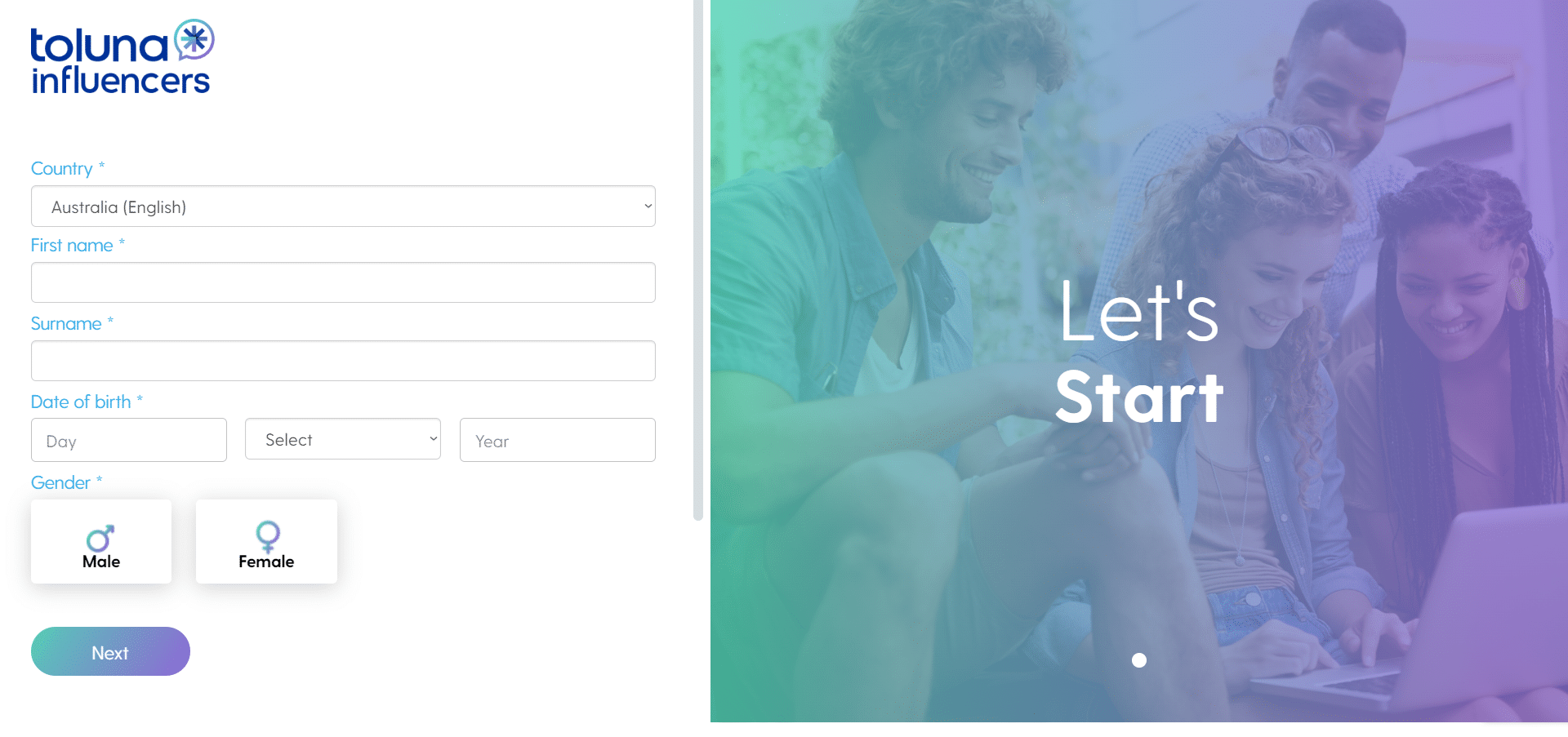This screenshot captures the sign-up page for the Toluna Influencers website. The layout features a split screen design. On the left side, there's a white background with various form fields for user information. These fields include categories such as "Country," defaulting to "Australia (English)," "First Name," "Surname," and "Date of Birth." The Date of Birth section is divided into three input areas for day, month selectable from a dropdown menu, and year. There is also a section for "Gender" which regrettably offers only "Male" and "Female" options. The text within these sections is a medium blue, while the input field borders are highlighted in medium gray.

Below the fields, there's a distinctive, rounded rectangular button adorned with a green-blue-purple gradient and white text reading "Next." 

On the right side of the screen, there's a welcoming header image featuring a diverse group of people, consisting of two men (one white, one black) and two women (one white, one black), gathered around a laptop held by the white woman. This image is overlaid on a green-purple gradient background, with the text "Let's Start" invitingly displayed at the top.